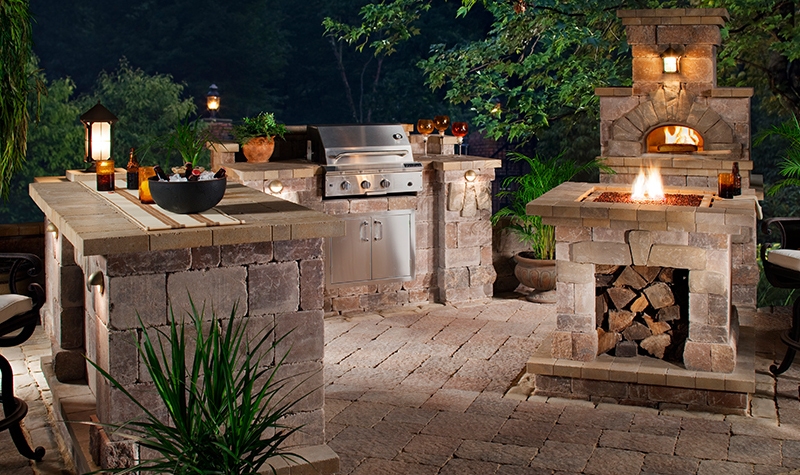This photograph captures an elaborate and inviting outdoor kitchen area, illuminated beautifully at nightfall. The entire setup is comprised of intricately detailed stonework. At the farthest part, a grill is integrated into a stone counter, which also features metal doors beneath it. Adjacent to this is a stone fire pit filled with logs, crackling with an active fire. Dominating the background is a stone pizza oven with what appears to be a loaf of bread or pizza inside. The scene is enhanced by abundant greenery, including thick trees behind the kitchen and potted leafy plants nearby, adding a touch of natural charm.

This nocturnal scene is brought to life by a variety of light sources: at least three lanterns and the glow from two fire features. The counters are adorned with bowls, possibly containing herbs or spices, and an array of glasses and champagne flutes, suggesting a lively atmosphere. Several chairs are pulled up to different sections of the bar, hinting at the presence of people. The entire setup exudes a sense of warmth and conviviality, epitomizing a perfect outdoor gathering spot.